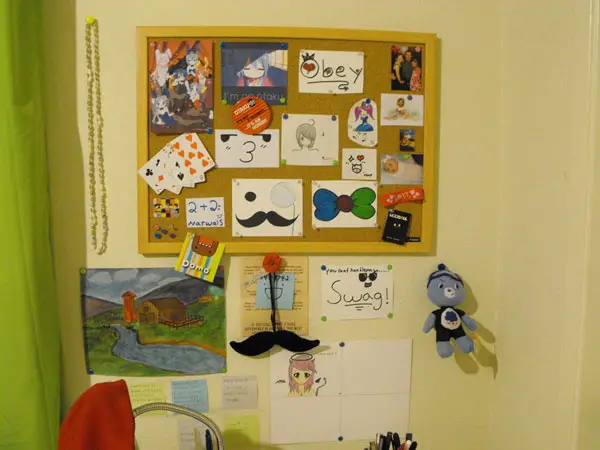The photograph depicts an indoor setting with a cream-colored wall adorned with various objects and decorations. Centered at the top is a yellow cork board filled with numerous pictures, stickers, and handmade drawings, including images of anime characters and some playing cards. Prominently featured on this board is a family photo in the top right, a mustache drawing with an eye and a monocle, and a title that reads "Obey." Below the cork board, a variety of items hang on the wall, such as a handmade scenery drawing of a river and barn, a blue plush doll resembling a bear, and a paper with "swag" written on it. To the left of the board, a large yellow push pin holds a dangling necklace, while a green curtain on the far left casts a shadow over the scene. The overall display, which also includes references to anime themes, suggests the personal touches of a young Japanese girl’s room.